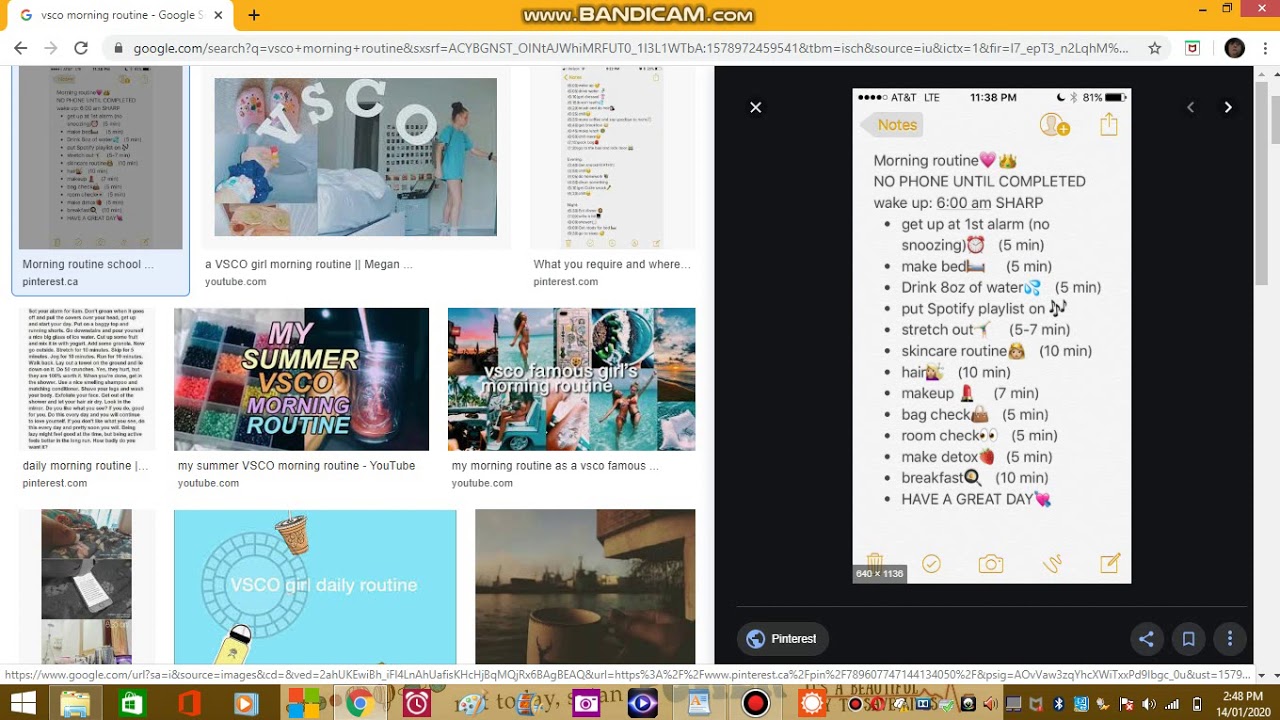The screenshot displays two open tabs on a computer screen. The prominent tab in focus is a Google search results page for "VSCO morning routine." The adjacent tab on the right is associated with www.bandicam.com, distinguished by a lengthy yellow banner running horizontally across the top.

The Google search results for "VSCO morning routine" list a variety of links:
1. Morning Routine School
2. VSCO Girl Morning Routine Megan
3. What You Require and Where
4. Daily Morning Routine
5. My Summer VSCO Morning Routine at YouTube
6. My Morning Routine as a VSCO Famous at YouTube

On the right side of the search page, a large black pop-up appears, displaying details from a Pinterest page. The text on the pop-up outlines a structured morning routine titled “Morning Routine: No Phone Until Completed.” The routine includes:

- Wake up at 6 AM sharp
- Get up at the first alarm, no snoozing for 5 minutes
- Make the bed in 5 minutes
- Drink 8 ounces of water within 5 minutes
- Put on a Spotify playlist
- Stretch out for 5-7 minutes
- Follow a skincare routine for 10 minutes
- Style hair in 10 minutes
- Apply makeup for 7 minutes
- Conduct a bag check taking 15 minutes
- Conduct a room check taking 5 minutes
- Prepare a detox beverage in 5 minutes
- Eat breakfast for 10 minutes
- Finally, "Have a great day!"

The image effectively captures the detailed sequence of a thematic VSCO morning routine search juxtaposed with another webpage related to Bandicam software.